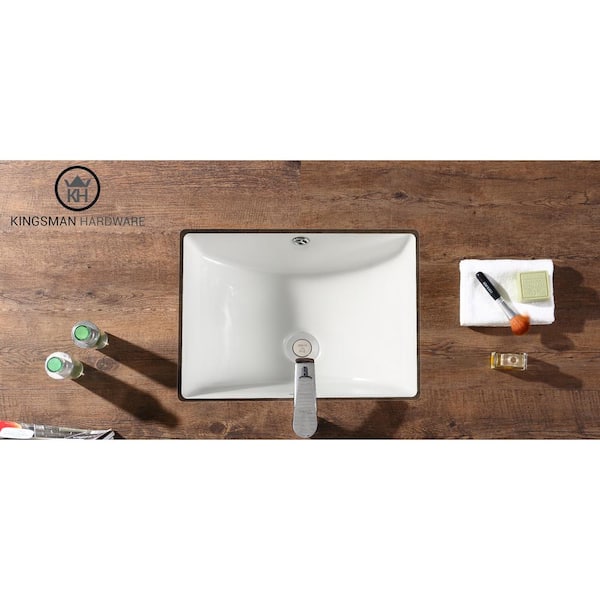The image showcases a pristine, porcelain white sink embedded in a dark brown wooden countertop, viewed from a top-down perspective. At the bottom center, the faucet nozzle is clearly visible. To the right of the sink, a makeup brush featuring an orange bristle head with a black handle and chrome midsection rests on a white towel, next to an indistinct box. On the left side, two glass bottles with green lids sit side by side. The upper left corner features a circular logo with a gray crown and the letters "K" and "H" in black, accompanied by the text "Kingsman Hardware." The overall composition hints at a neat, possibly computer-generated, advertisement for a product on a website.